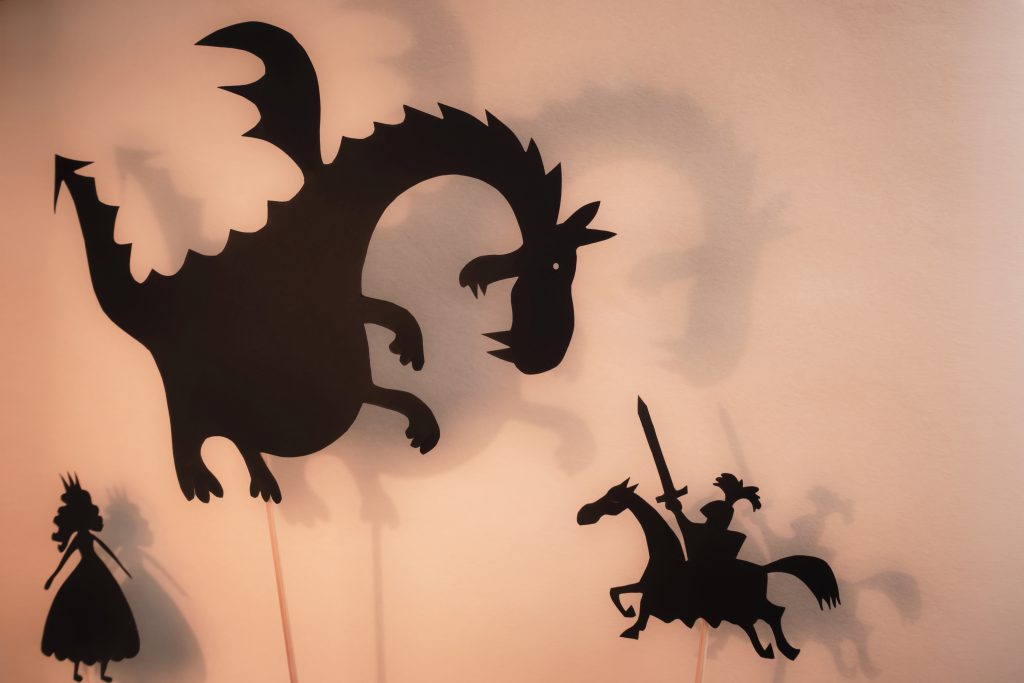The image is a computer-generated, cartoon-style depiction of a shadow puppet show. Set against a light tan or peach background, the scene is entirely rendered in black silhouettes. In the left-hand corner, there is a princess with long hair and a crown, clad in a dress that flares out like an upside-down wine glass. Her hands are spread apart, and she looks upwards at a dragon hovering in the air. The dragon is portly with a protruding belly, short legs, a long curved neck, wings flapping, and a tail sticking out.

Towards the right, a knight on a horse confronts the dragon. The knight is distinguished by a helmet adorned with feathers, an outstretched arm wielding a sword, and a shield in his other hand. The knight's horse, covered with a blanket that has a jagged bottom edge, stands boldly facing the dragon. Wooden sticks supporting each figure emphasize the puppetry aesthetic, with all elements casting soft shadows on the background wall. The scene captures a classic chivalric battle, complete with a damsel in distress, evoking the timeless tale of bravery and mythical creatures.